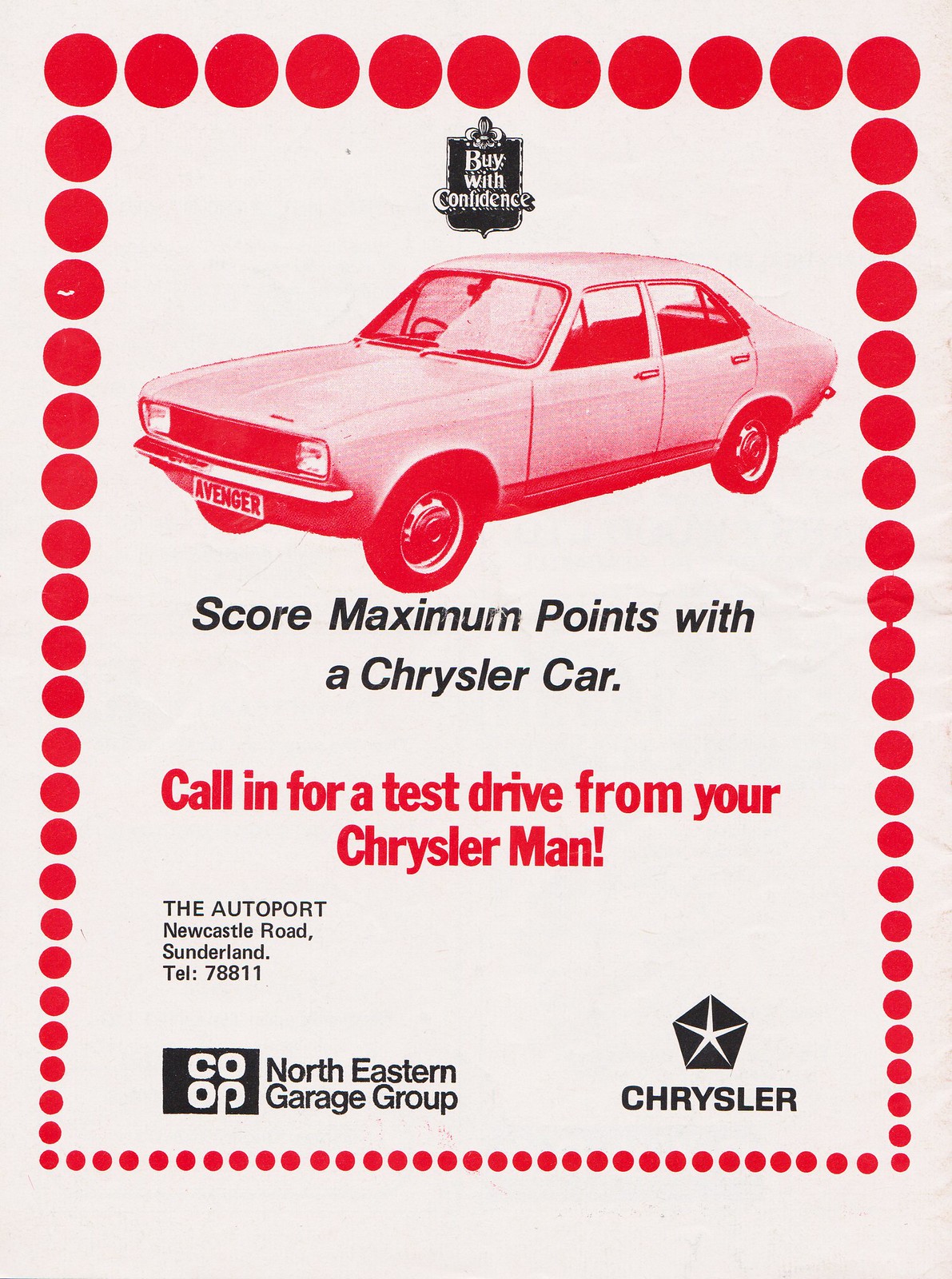This vintage advertisement flyer features a classic 1960s red car, presented on a white background with possible aged tones of grey or pink. The ad is bordered by a series of red dots, which gradually decrease in size from the top to the bottom, creating a dynamic frame. Centrally placed is the striking image of the red-tinted car with the license tag "Avenger." At the top of the car is a prominent shield-shaped emblem with the phrase "BUY WITH CONFIDENCE" in bold white letters. Below the car, the ad proudly states "Score maximum points with a Chrysler car" in striking letters, followed by "Call in for a test drive from your Chrysler man" in bold red font. Additional details include the address "The Auto Port, Newcastle Road, Sunderland, TELL 78811," with logos for the Northeastern Garage Corp in the bottom left and Chrysler in the bottom right. The color scheme is strictly composed of black, red, and white hues.